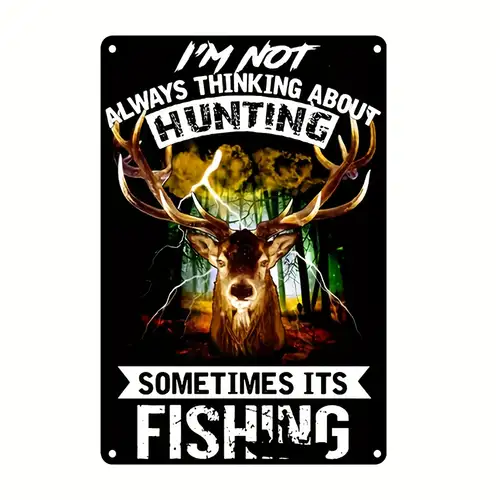This image features a detailed metal placard designed as a vertical rectangular sign with rounded corners and four holes, one in each corner, suggesting it can be nailed up. The sign has a predominantly black background with white text arched at the top that reads, "I'm not always thinking about hunting." The word "hunting" is displayed in black within an arched white border. Below, a white ribbon bar features black text reading, "sometimes it's," leading to the word "fishing," prominently displayed in white underneath. The "ing" in "fishing" cleverly incorporates a silhouette of a man standing on a small fishing boat. The center of the sign showcases a striking image of a deer with large antlers, staring straight ahead, with a dramatic forest and lightning storm serving as the background.